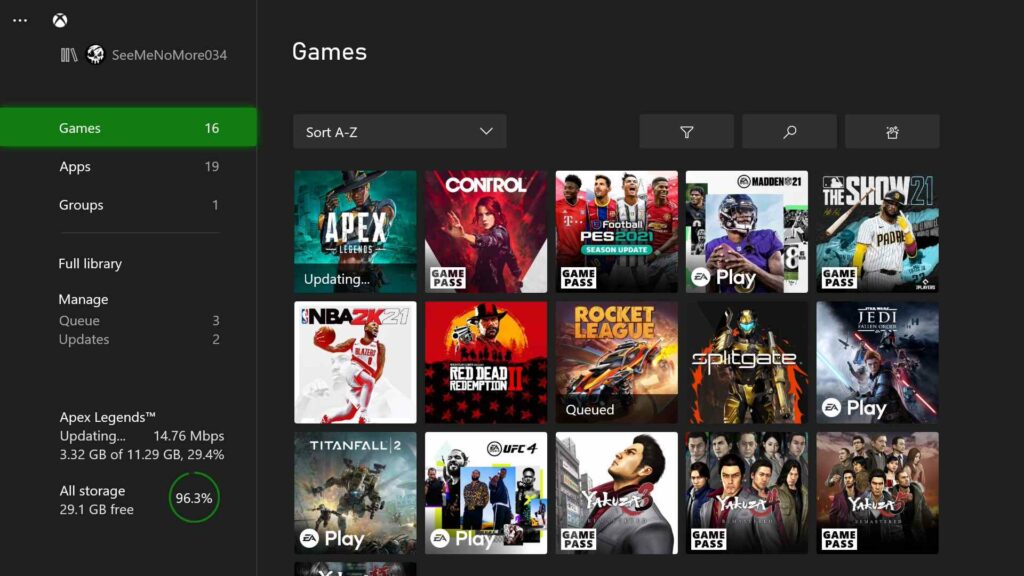The image depicts a web interface designed to display numerous clickable game options within a dark-themed layout. At the top of the interface, within a black rectangle, there is a white circular icon with an 'X' in the center, its function unspecified. Below this icon, the text "See Me No More 033034" is presented in a grayish font. Adjacent to this text on the right, the word "Games" is featured prominently in white.

The left column is primarily informational and exhibits various categories and statistics: 
- "Games" (16 items), highlighted in green
- "Apps" (19 items)
- "Groups" (1 item)
- "Full Library"
- "Managed Queue" 
- "Updates" (2 items)

Additionally, "Apex Legends™" is currently updating, downloading at a speed of 14.76 MBps, with 3.32 GB out of 11.29 GB completed (29.4%). The storage information indicates 29.1 GB is free.

A green circular icon displays "96.3%".

The main section of the interface lists games in a 4x3 grid:
1. Apex
2. Control
3. Past 2021
4. Madden (assumed)
5. The Show
6. NBA 2K21
7. Red Dead Redemption
8. Rocket League
9. Splitgate
10. Jedi
11. Titanfall
12. UFC

The final three game titles appear to be in another language, which is not specified.